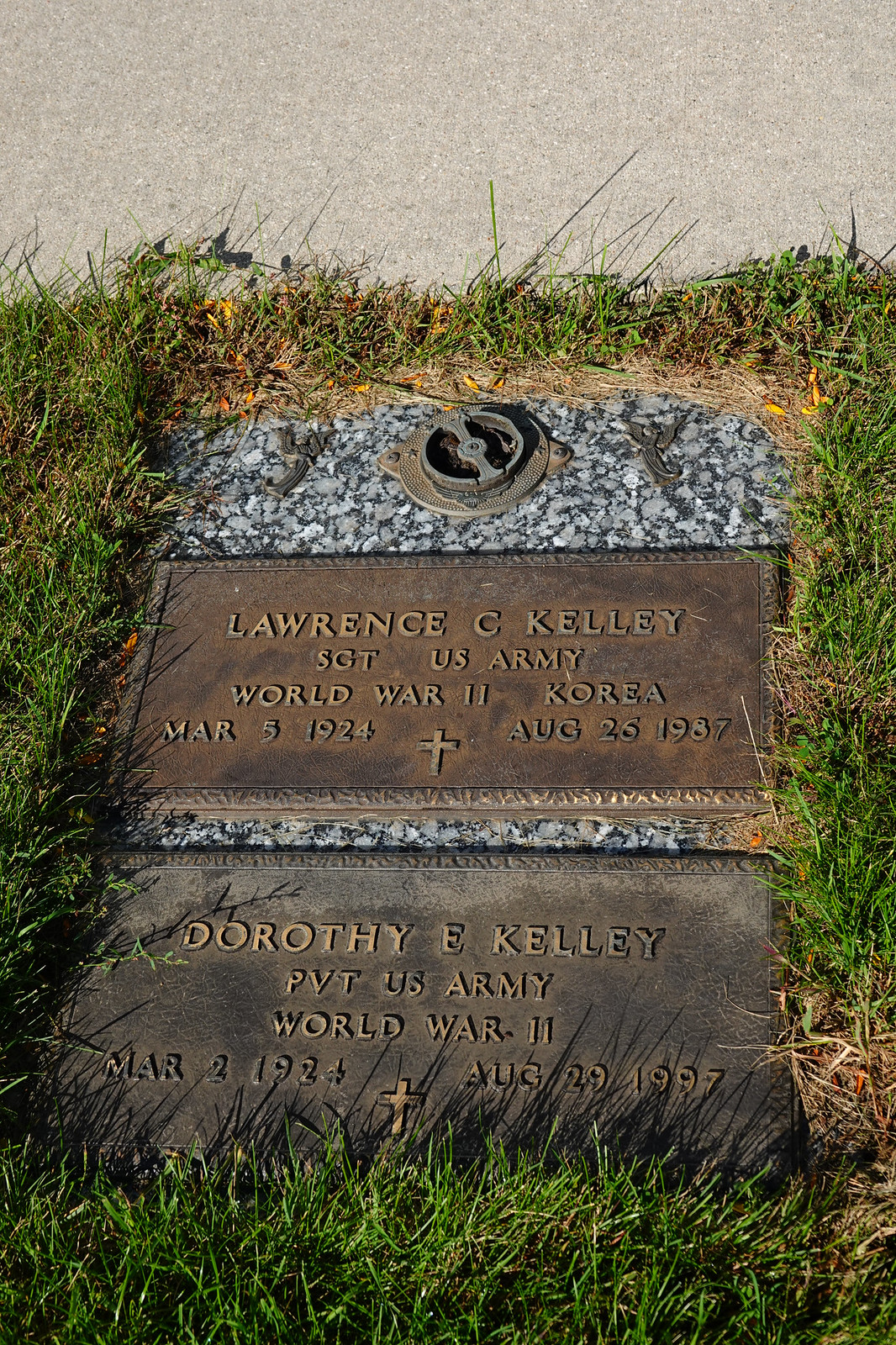This image depicts a grave featuring two bronze nameplates set in brown stone gravemarkers, surrounded by lush green grass. The top nameplate reads: "Lawrence C. Kelly, Sergeant, U.S. Army, World War II, Korea, March 5, 1924 - August 26, 1987," and it is adorned with a Christian cross in between the dates. Below it, the second nameplate reads: "Dorothy E. Kelly, Private, U.S. Army, World War II, March 2, 1924 - August 29, 1997," also featuring a Christian cross between the dates. Flanking the nameplates, on either side, are ornamental bird-like designs or angel emblems, and above the plates, a circular metal aperture is affixed to the gravemarker. Mixed pebbles are scattered around the stones, adding texture to the scene, with a stone-gray pavement situated just above the grave.